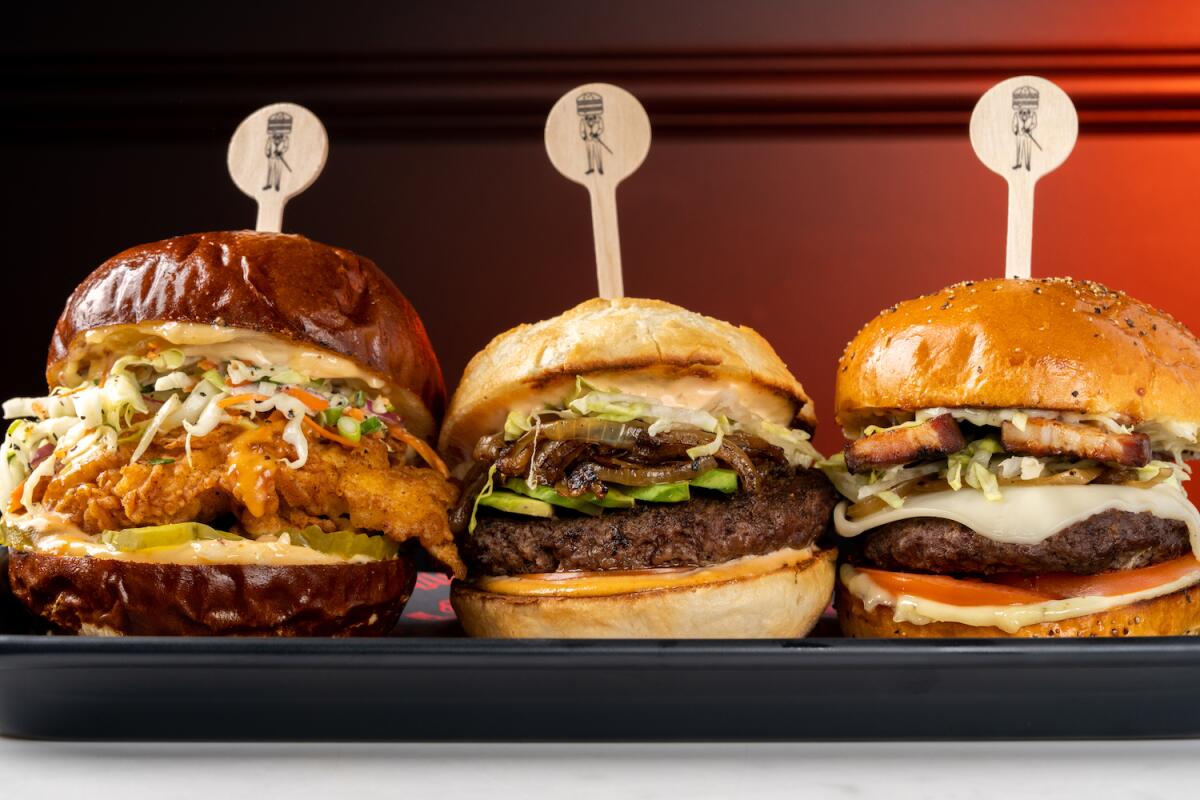The image showcases three sandwiches, each distinct in its presentation, arranged on a black tray against a red background. The sandwich on the left features a crispy, breaded chicken or fish patty encased in a dark, pretzel-like bun, complemented by coleslaw, finely cut cabbage, carrots, and possibly cucumbers. It's topped with a figure of a man on a circular toothpick. The middle sandwich, slightly smaller, has a lighter-colored bun and reveals a hamburger with layers that include mayonnaise, pickles, lettuce, onions, and potentially avocado. The sandwich on the right is the largest, with a medium-brown bun and contains a cheeseburger with white cheese, an array of condiments, lettuce, mayonnaise, and a hint of tomato. All three sandwiches are adorned with the same distinctive toothpick featuring a circular top with a human figure image.